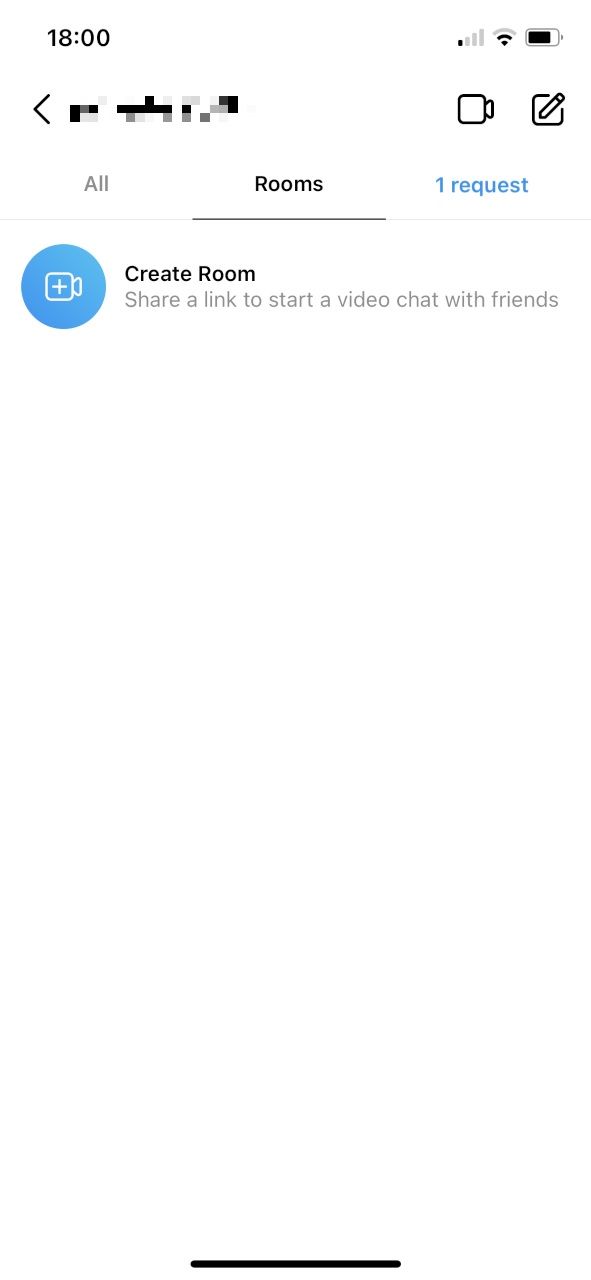In this image, a smartphone screen displays an app interface for video chatting. The top of the screen features a typical phone header showing the time as 18:00, a Wi-Fi connectivity icon, and a nearly full battery indicator. Below the header, a back arrow suggests the user is within a submenu. Any text to the right of this arrow is blurred and indistinguishable. Adjacent to this blurred text is a camera icon, followed by a pencil icon enclosed in a square, likely indicating an editing function.

Further down, the interface lists three subpages, the titles of which appear as "All," "Rooms," and "Requests." The "Rooms" tab is highlighted in dark black with an underline, indicating it is the currently selected page. This suggests it is where users can create or join chat rooms to communicate with friends.